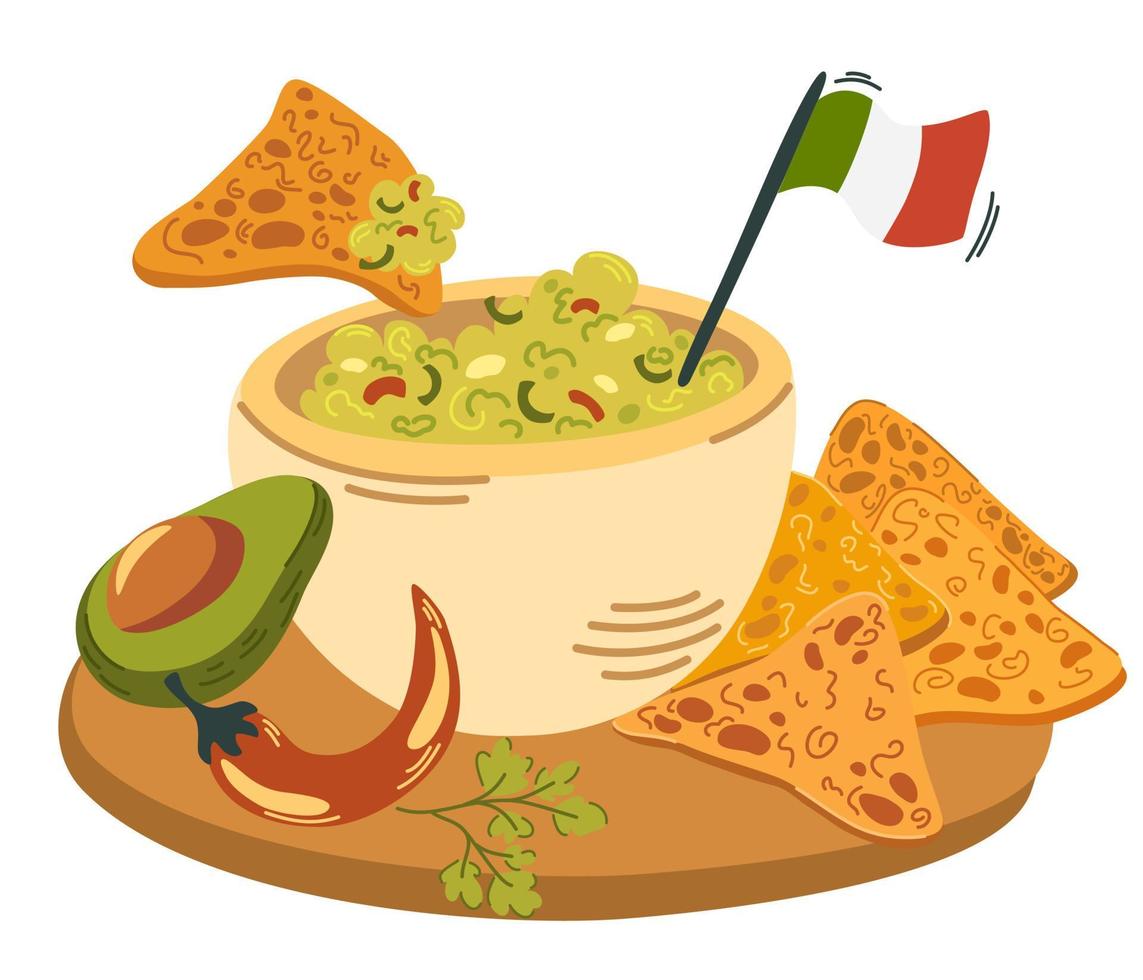The illustration depicts a tan bowl brimming with green guacamole, accentuated by visible pieces of red and green peppers, and sitting on a circular brown tray that resembles a cutting board. The guacamole is garnished with a small flag—most likely the Mexican flag, displaying green, white, and red vertical stripes—from a stick emerging from the bowl. Surrounding the bowl are various elements enhancing the scene: on the left side of the tray, a half-cut avocado with its seed intact, a red chili pepper, and some parsley garnish. To the right, there are a handful of large tortilla chips, with one chip illustrated floating above the bowl, dipping into the creamy guacamole.